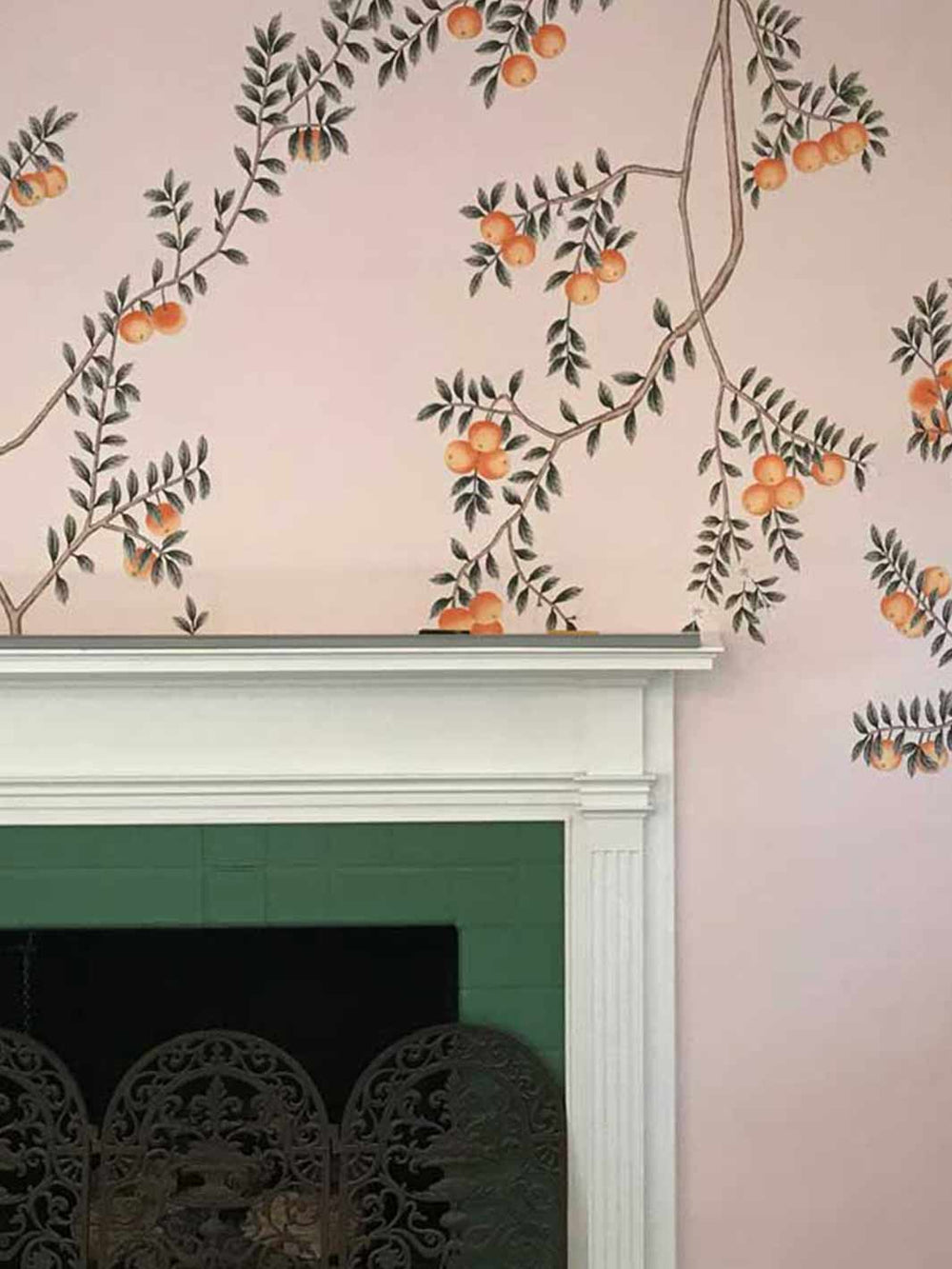This indoor photograph, captured in portrait orientation, features a prominently displayed fireplace mantel situated slightly to the left of the center. The white wooden mantel with raised molding, extending down the sides and trimmed across the top, frames the scene. Below, the fireplace is encased with green-painted brick, leading to a dark interior containing a few pieces of stacked wood. In front of the fireplace, there's an ornate black wrought-iron screen, designed with arched panels for an aesthetic appeal.
 
The wall above the mantel is covered in a light pink wallpaper that dominates the upper portion of the image. This wallpaper is intricately decorated with numerous tree branches adorned with small, dark green leaves. Emerging from these branches are clusters of orange-hued fruits, perhaps peaches or similar, adding a vibrant and lively touch to the backdrop. The wall’s artwork, reminiscent of a garden in full bloom, accentuates the warm, welcoming ambiance of the room. The photograph's style reflects a realistic, representational approach, capturing detailed elements of the fireplace and its surroundings.